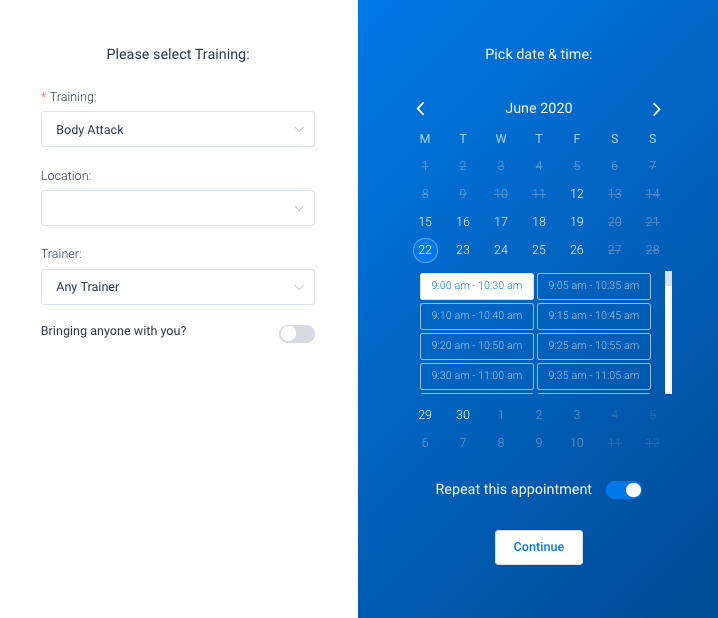The image depicts a comprehensive interface for booking a training appointment. The screen is divided into two sections, each with a distinct color scheme. On the left side, which has a white background with black text, users are prompted to select their training preferences. The heading "Please Select Training" is accompanied by an asterisk, indicating a required field. A drop-down box labeled "Training" is currently set to 'Body Attack,' and another drop-down box for "Location" shows no selection. Additionally, under the "Trainer" section, 'Any Trainer' is pre-selected. There is also a question, "Bringing anyone with you?" followed by a toggle switch allowing users to indicate yes or no.

The right side of the screen features a medium dark blue gradient background with white text. It is dedicated to choosing the date and time for the appointment. The calendar is set to June 2020, and the user has selected Monday, the 22nd. The chosen time slot is from 9:00 AM to 10:30 AM. Below this, a toggle switch allows users to set the appointment to repeat. This option is currently activated as indicated by the toggle being switched on. At the bottom center of the blue section, a prominent white button with blue text reads "Continue," inviting the user to proceed with their booking.

Every detail on this interface is clearly organized to facilitate the user’s training appointment scheduling, highlighting selections and required fields efficiently.